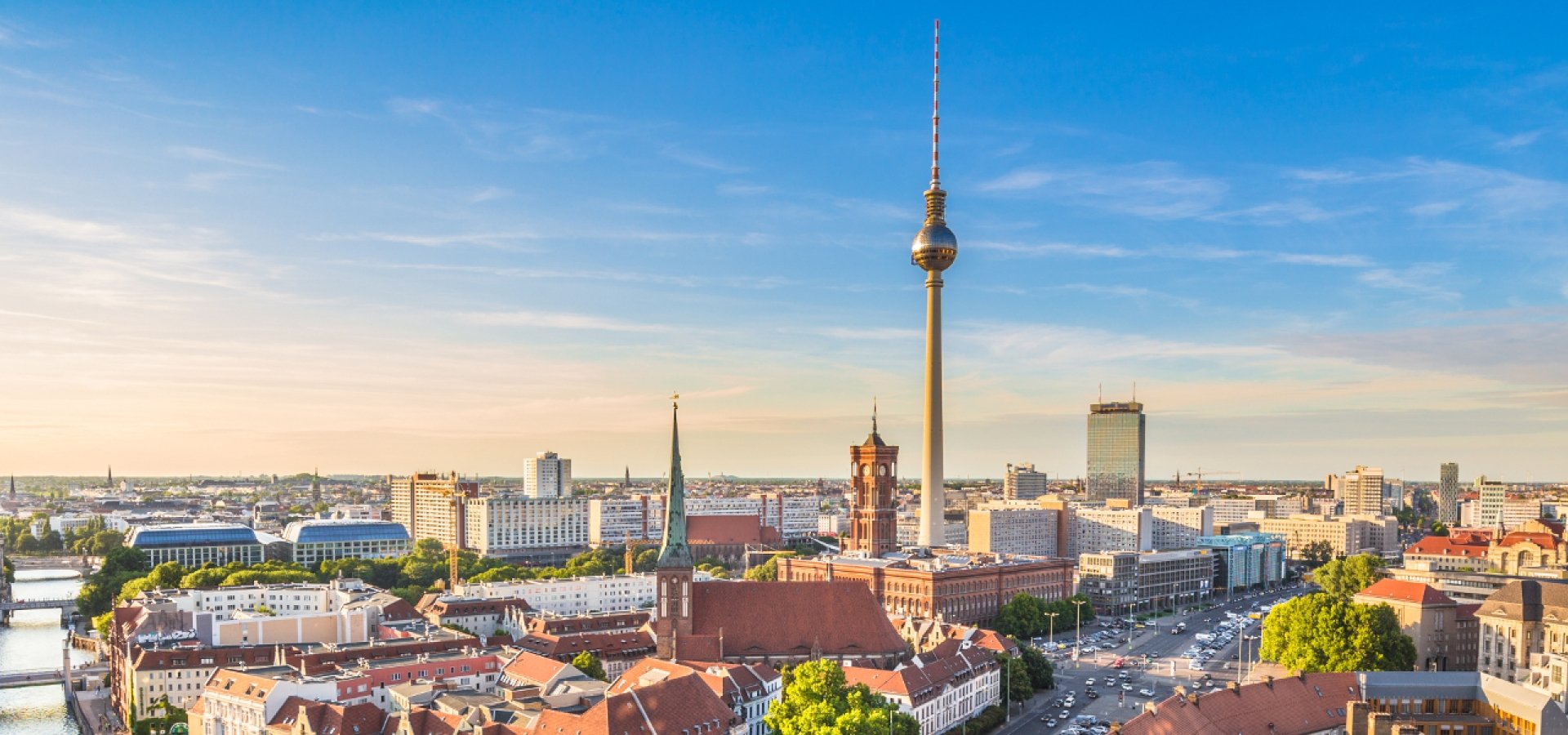The image captures a vibrant cityscape featuring a diverse array of buildings, each showcasing different colors, structures, and architectural styles. A prominent road stretches from the bottom left to the bottom right corner, busy with moving cars and spanning three to four lanes. Rooflines are visible at a treetop level, enhancing the depth of the scene, while a clear sky—partly cloudy with beautiful blue hues—suggests the photo was taken during the day, possibly at dawn or dusk.

Dominating the center of the city is a soaring, pointy skyscraper that stands out distinctly from the rest. This towering structure starts with a concrete base and transitions into a more metallic appearance as it ascends. Topping the skyscraper is a metallic ball, followed by a sharp, red-tipped spire decorated with red and white stripes, resembling the iconic Space Needle but unique in its details. The overall perspective suggests the photo was taken from an elevated vantage point, providing a clear and expansive view of the skyline that extends far into the horizon.